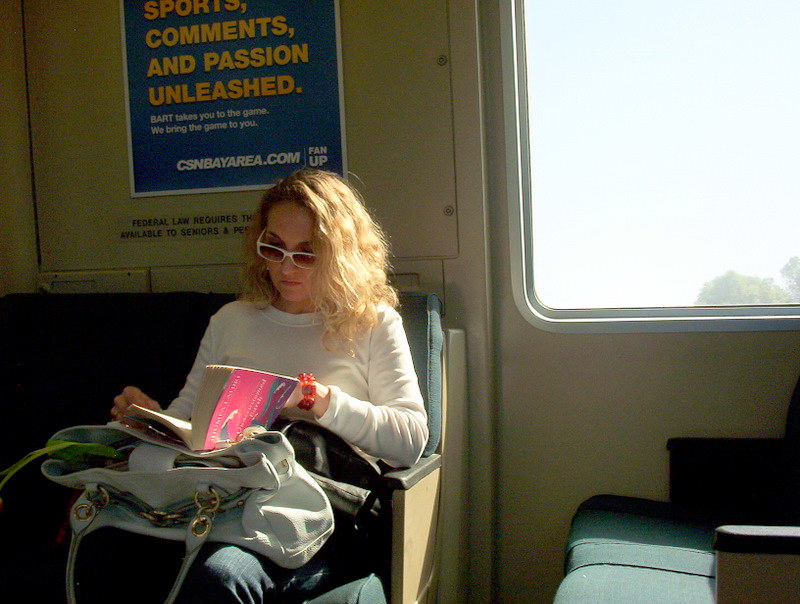A woman is sitting on a seat in a subway car, facing the window. She has wavy blonde hair and is dressed in a long-sleeved white top and blue jeans. She accessorizes with a red bracelet on her wrist and white-framed sunglasses perched on her head. In her hands, she is engrossed in a book with a vibrant pink, blue, and purple cover. Her gray purse and a dark-colored jacket rest on her lap. The seats in the subway car are teal with matching cushions, and the frame of the seats is tan with gray armrests. In the background, a blue poster with yellow and white text is visible, along with a window that looks out onto the surroundings.